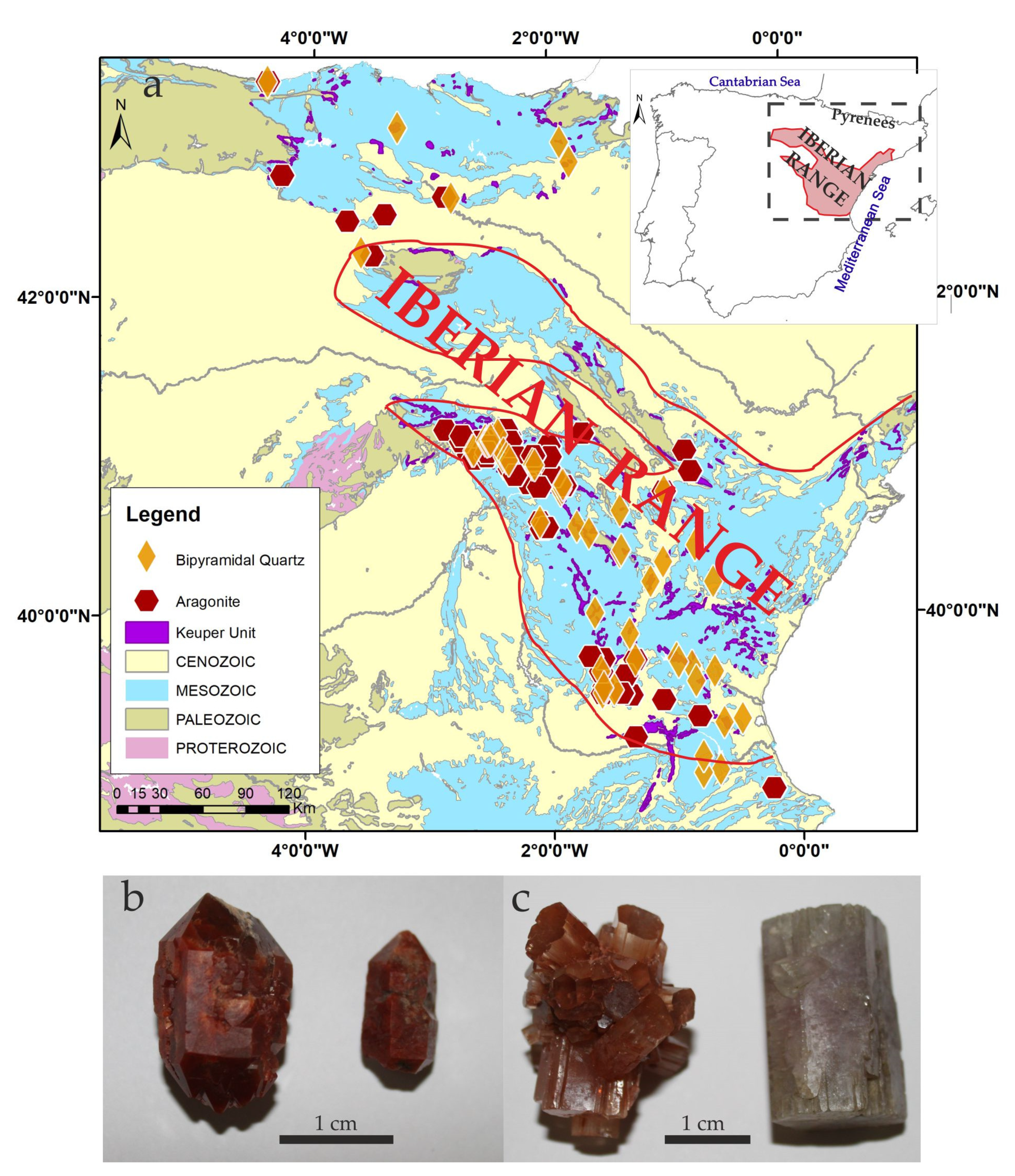The image is a comprehensive display featuring the geological and mineral map of the Iberian Range in Spain and photographs of crystals found in this region. The top two-thirds of the image is dominated by a detailed map of the Iberian Peninsula with specific points of latitude and longitude, highlighting the Iberian Range. A smaller inset in the upper corner shows the location of the Iberian Range within the broader context of Spain. The map includes a legend with various colors indicating different mineral deposits, including bipyramidal quartz and aggreganate. 

Several regions within the Iberian Range are circled and marked, indicating where these minerals and crystals can be found. The map also features information about the geological history and soil deposits in these areas. 

At the bottom of the image, there are four photographs of crystals, each compared to a one-centimeter scale to emphasize their small size. Three of these crystals exhibit a brown or copper hue, while the fourth has a silver, more metallic appearance. The crystals, described as cylindrical and aggregated, include types like bipyramidal quartz and argonite, corresponding to those indicated on the map.